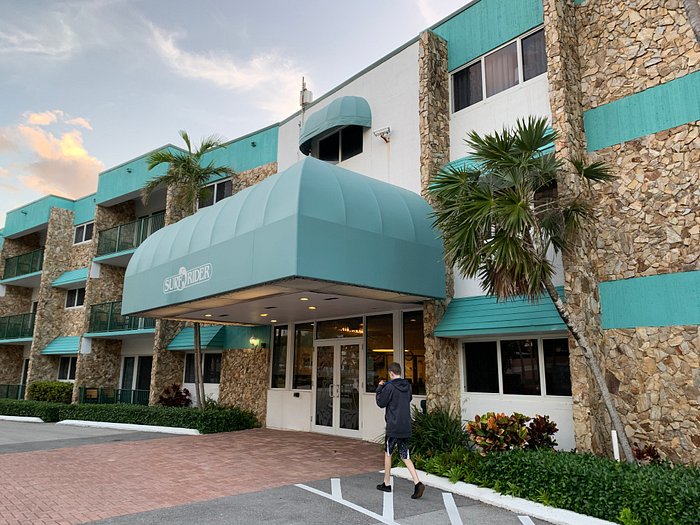This photo captures the front view of a three-story hotel, identified as "Surf Rider," during the daytime. The building's facade features a combination of white walls and brown stones, creating a striped pattern. The central entrance is marked by a prominent green awning that bears the hotel's name. Above the first-floor patio and extending across the second and third floors are balconies. 

The left section of the building is characterized by a protruding stone column and green bands at the top and bottom of a stone wall. In front of this wall, a tree with green branches bends slightly to the left. To the far right of the image, the white curb borders green bushes adding to the greenery and leading toward the hotel's entrance.

A young man, possibly a teenager, dressed in black shorts with white stripes, black sneakers, and a black hoodie, walks along a gray pathway with white markings towards the entrance. The ground leading up to the entrance comprises reddish stone paving, with an adjacent asphalt driveway. There is no vehicular traffic visible, suggesting a peaceful and quiet setting.

In the background, a blue sky with patches of orange-tinged clouds indicates it's early morning. The leftmost part of the building extends out of the frame, but visible sections show additional balconies and more stone and white walls.